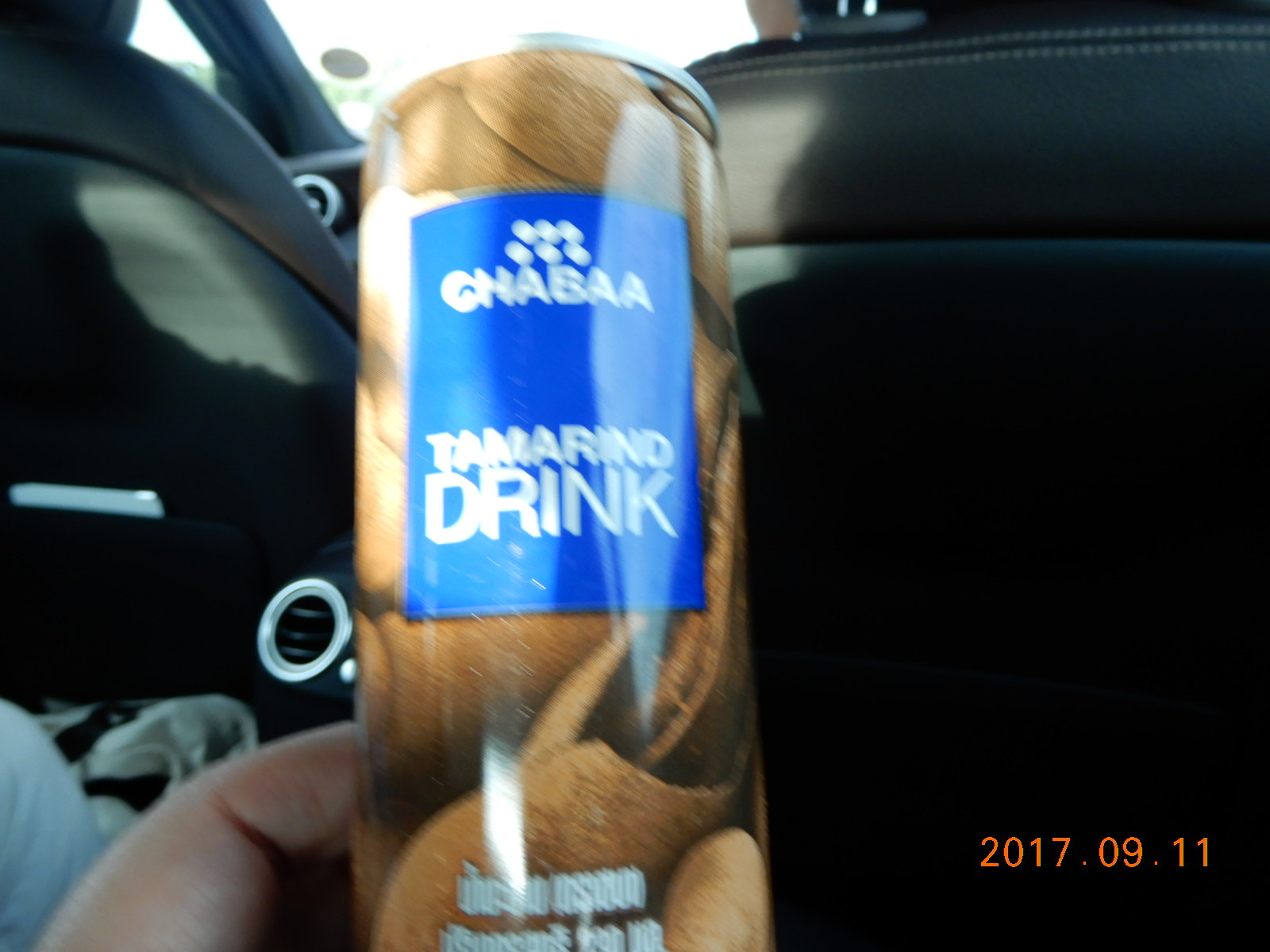This image, taken on September 11th, 2017 from the back passenger seat of a car, features a close-up of a tall can of GABA Tamarind (or Tamarino) drink. The left hand of a light-skinned individual holding the can is visible, along with part of their leg clad in greenish-gray pants. The can, displaying a dark blue label with white lettering and some brown leaf designs, is slightly tilted to showcase the label which prominently reads "GABA Tamarino drink." The photograph, which appears to be slightly blurred, shows the car's interior with black upholstery and dark gray or possibly black leather front seats. Two air conditioning vents are visible—one in the back seat near the hand holding the can and another at the front near the windshield. The windshield itself reveals a bright, sunlit sky outside. The image includes a date stamp at the lower right corner indicating it was taken on a digital camera on September 11th, 2017.